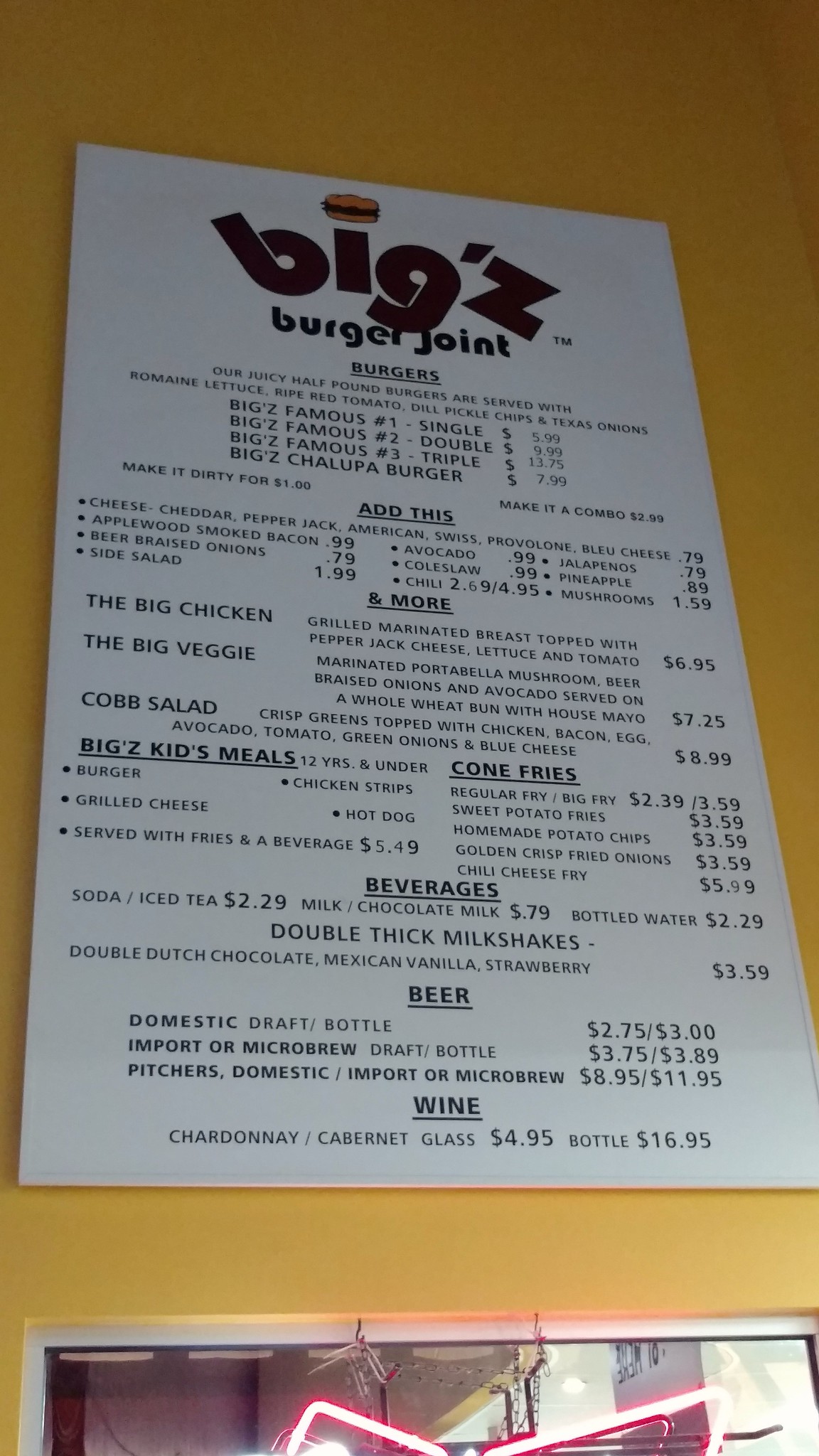This photograph captures the detailed wall menu of "Bigg'z Burger Joint," a popular eatery known for its extensive offerings. The menu, a white rectangular board with brown lettering, is prominently mounted on a vibrant yellow painted wall. Below the main menu, the top part of a neon beer sign is visible, reflected in a way that hints at it being a Budweiser logo.

The menu is meticulously sectioned to guide customers through its variety. It begins with the signature "Famous Number One Single" burgers, followed by options for double and triple patties. Guests can choose to "make it dirty" or opt for a combo meal. The "Add This" section provides customization options, including different cheeses, side salads, and coleslaw, to enhance the burger experience.

Adjacent to this is the "& More" section, featuring a range of additional items such as chicken, veggie sandwiches, and a Cobb salad. For the younger patrons, the "Bigg'z Kids Meals" offers kid-friendly options. The menu also includes a unique item labeled "Cone Fries" and an assortment of beverages. Patrons can choose from draft or bottled beer, with wine options limited to either Chardonnay or Cabernet, ensuring a complementary drink for any meal choice.

The detailed menu highlights the diverse offerings of Bigg'z Burger Joint, appealing to a wide range of tastes and preferences.